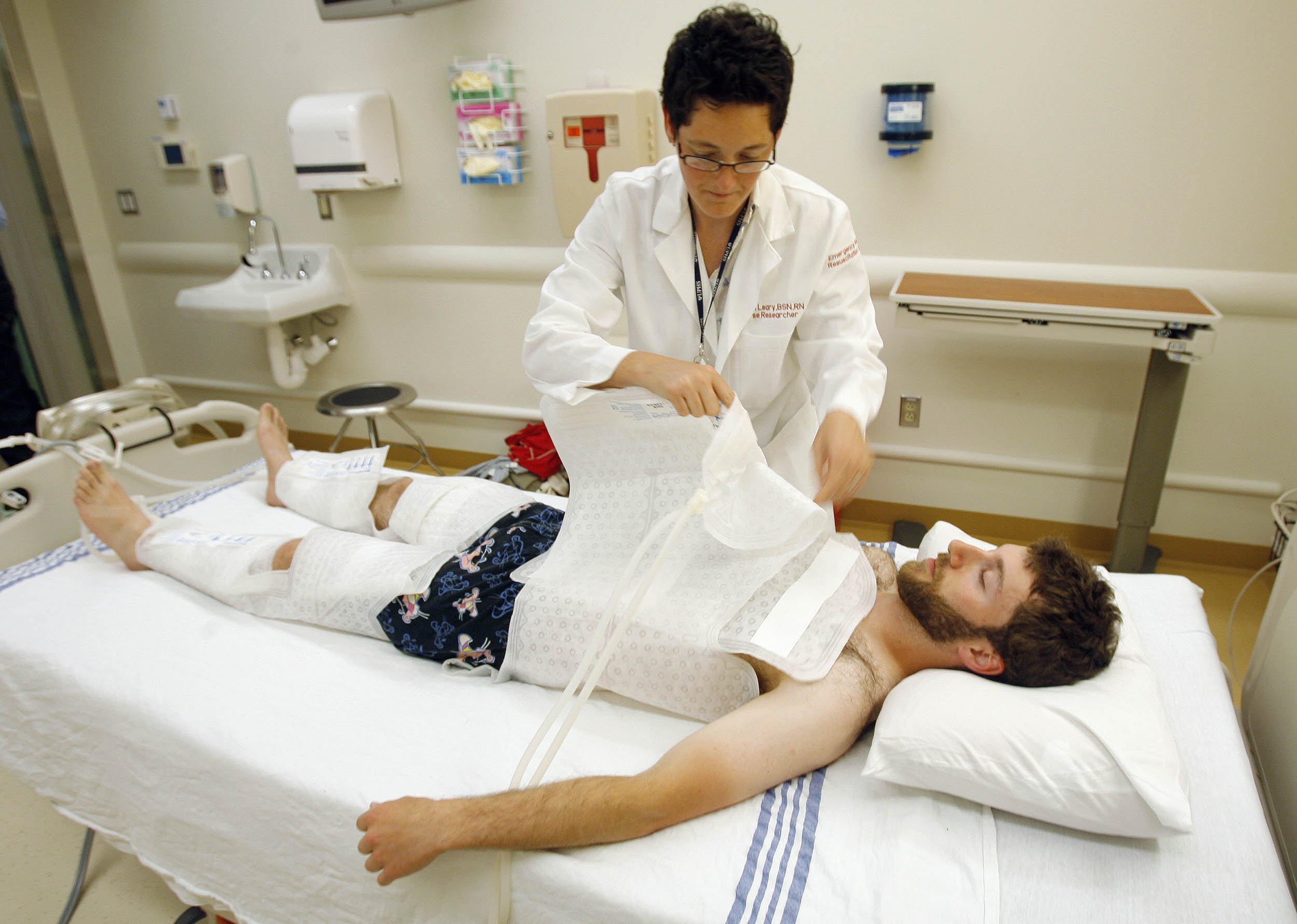A detailed side-angle view photograph captures a young man, likely in his late 20s to early 30s, lying on a hospital bed with a white fluffy pillow under his head. He is wearing blue shorts adorned with a pink swirly pattern. The man has dark brown hair, a goatee, and a beard, and his expression appears somewhat dazed. His legs are extensively wrapped in gauze and white flexible fabric, extending from his ankles to above his knees. Similarly, his chest is wrapped in a fluffy material with ties protruding from the top. 

Hovering over him is a female doctor, distinguished by her short dark brown hair, white lab coat with white lettering over the right breast pocket, and red writing on the upper right sleeve. She also wears glasses and a lanyard, seemingly focusing on his chest as she applies bandages.

The hospital room setting is depicted with a white background wall adorned with various medical essentials. To the left, a needle collection box, a white shelf with different glove boxes, a sink, a paper towel dispenser, and a hand sanitizer dispenser are meticulously arranged. On the right side of the image, an adjustable table with a brown top is pushed against the wall, contributing to the clinical environment. A small table for medical instruments and a stool are also visible, enhancing the sense of a functional medical treatment space. The arrangement and items in the room suggest a typical hospital or clinical setting, possibly reflecting post-surgery care or treatment for an injury.